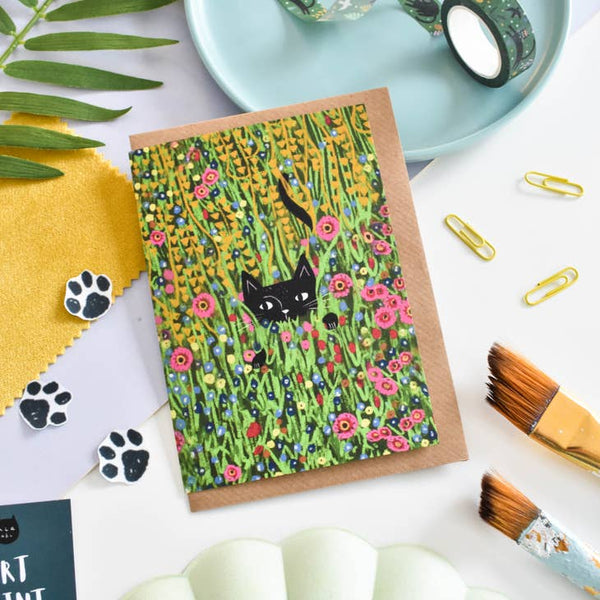This image depicts a detailed, hand-painted greeting card, featuring a black cat amidst an array of tall, vibrant flowers. The card, approximately the size of a traditional envelope insert, is partially askew and underlines artistic creativity. The cat is surrounded by a lush garden of pink and yellow blossoms, while various art supplies are scattered around. On the bottom right, two angled paintbrushes rest on the white surface, above which lie three yellow paper clips. To the left, a cutout of three black cat paws adds a playful touch. Adding to the scene's complexity, the top left corner of the image reveals a stem with leaves, and just to its right, a pale blue plate holding what appears to be tape rolls. The overall composition suggests an engaging and whimsical workspace, potentially for crafting greeting cards or indulging in creative projects.